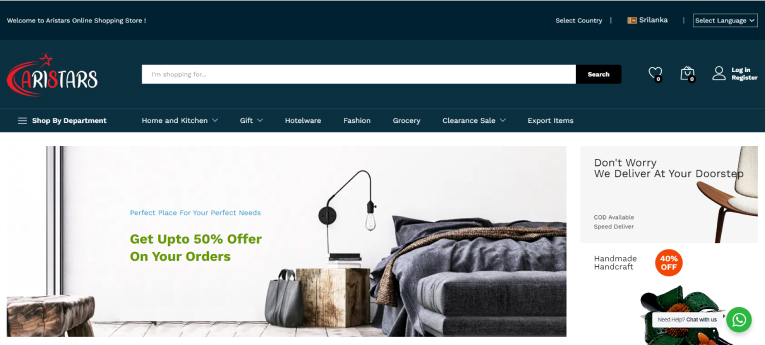This image depicts a webpage from the Airstars Online Shopping Store. The webpage features a predominantly white background with a prominent blue navigation bar at the top. The blue bar includes white text and a few colorful icons, enhancing the visual appeal. The rest of the page is primarily adorned with various pictures against the white backdrop.

At the top of the page, a welcoming message reads, "Welcome to Airstars Online Shopping Store," accompanied by options to select the country (Sri Lanka) and language. On the left side, there's a red and white logo reading "Kari Stars," with a star replacing the letter "I."

Below the logo, a search box prompts users with the text "I'm searching for," accompanied by a search button. To the right of the search box are icons representing a heart (likely for favorites), a bag (presumably for the shopping cart), a user icon, and a login button.

The main content area features several images: 

1. A photograph showcasing a bedroom with a bed and a lamp, overlaid with the text, "Perfect place for your perfect needs. Get up to 50% offer on your orders."
2. To the right, another image with the text, "Don't worry, we deliver at your doorstep. COD Available, Speed Deliver."
3. An additional image advertises "Handmade Handcraft, 40% off."

A WhatsApp chat button at the bottom-right corner offers assistance with the text, "Need help? Chat with us."

At the top of the page, further navigation options are available, including categories like Home and Kitchen, Gift, Hotel World, Fashion, Grocery, and Clearance Sale. The overall layout suggests Airstars is an online retailer specializing in a variety of products, with a focus on furniture and home goods.